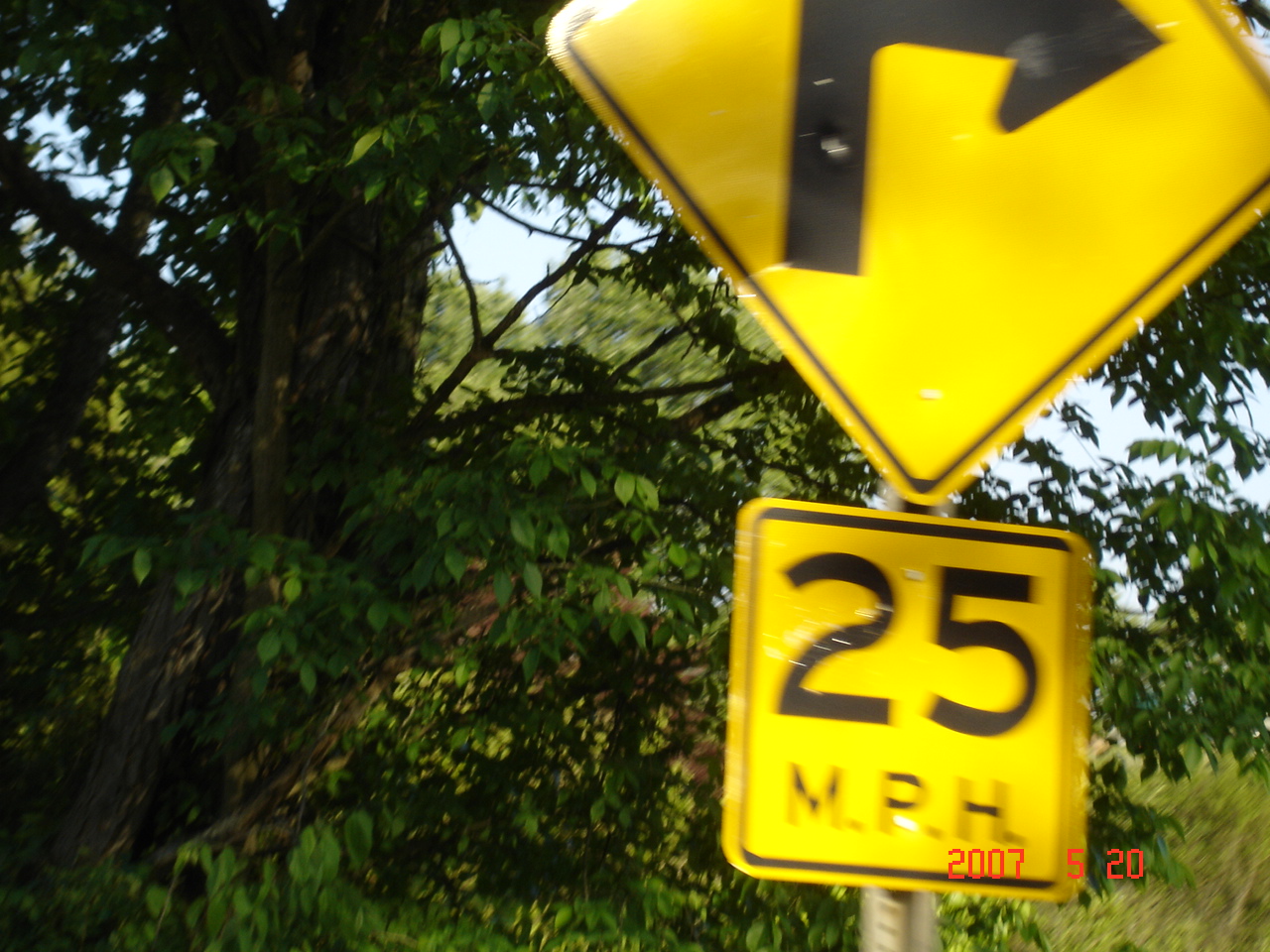This landscape photo, taken during the daytime, features a bright yellow diamond-shaped road sign on the right edge of the frame. The sign prominently displays a right turn symbol, with a supplementary placard below it indicating a safe speed of 25 miles per hour. The road sign is positioned up close in the foreground and appears slightly out of focus, directing attention to the lush, green background. In the background, a dense array of trees and underbrush is visible, hinting at an overgrown, natural area. Among these trees, one large, mature tree stands out against the smaller, verdant foliage. The highway to which this sign likely pertains is not visible in the photograph.